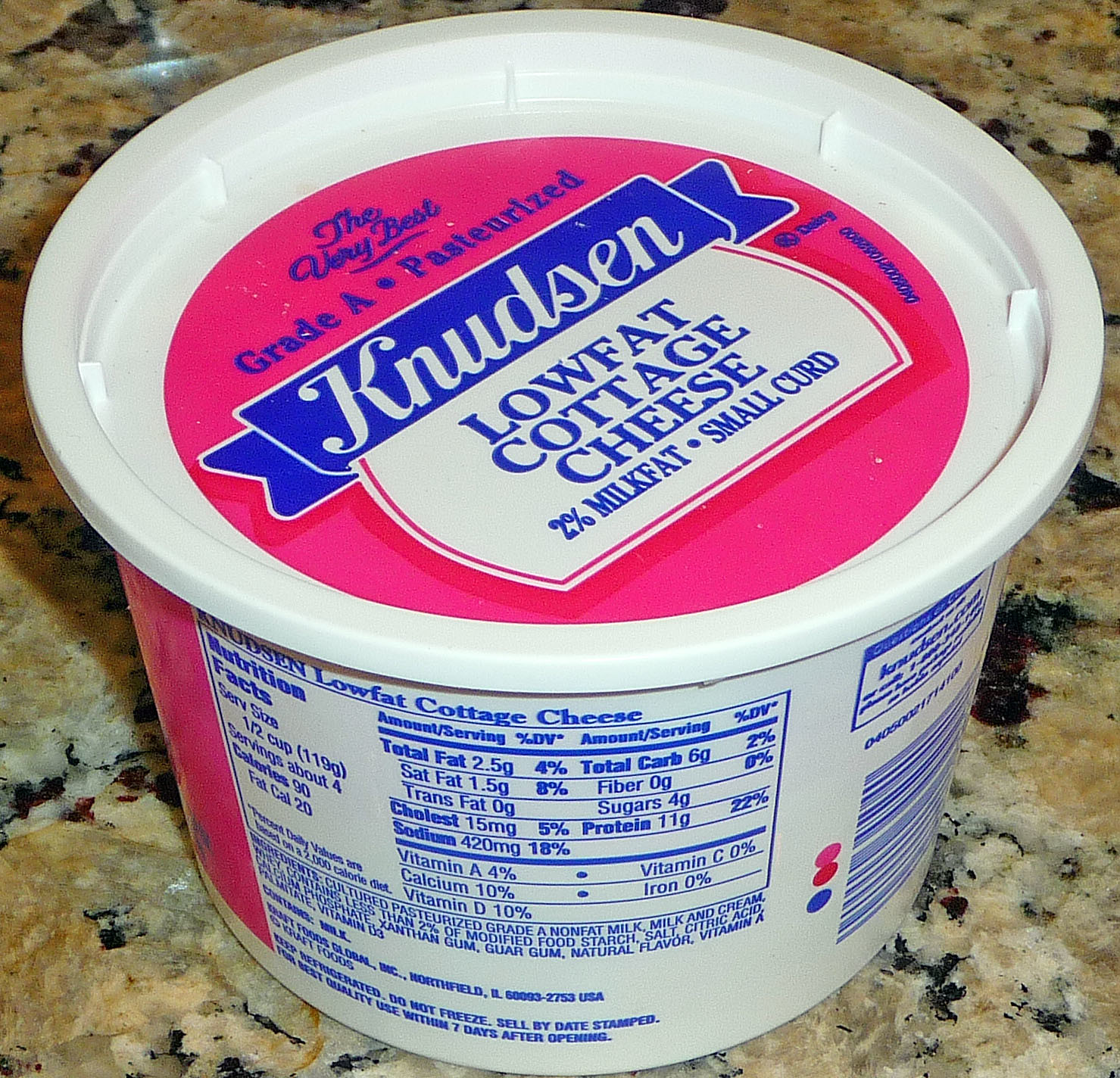A small tub of Knudsen low-fat cottage cheese is prominently displayed on a marble countertop featuring a blend of black, beige, and white hues. The tub itself is predominantly white with a distinctive pink circular label. The brand name, "Knudsen," is prominently printed in white letters set against a blue ribbon background. The description "low-fat cottage cheese" is written in blue letters on a white field, with additional text below stating "2% milk fat, small curd," also in blue lettering. Above the brand name, the phrase "the very best grade A pasteurized" is inscribed in blue. The photo captures the tub from a top-angle perspective, offering a clear view of the side, which displays the nutrition facts: 2.5 grams of fat, 420 milligrams of sodium, and 11 grams of protein, among other details.